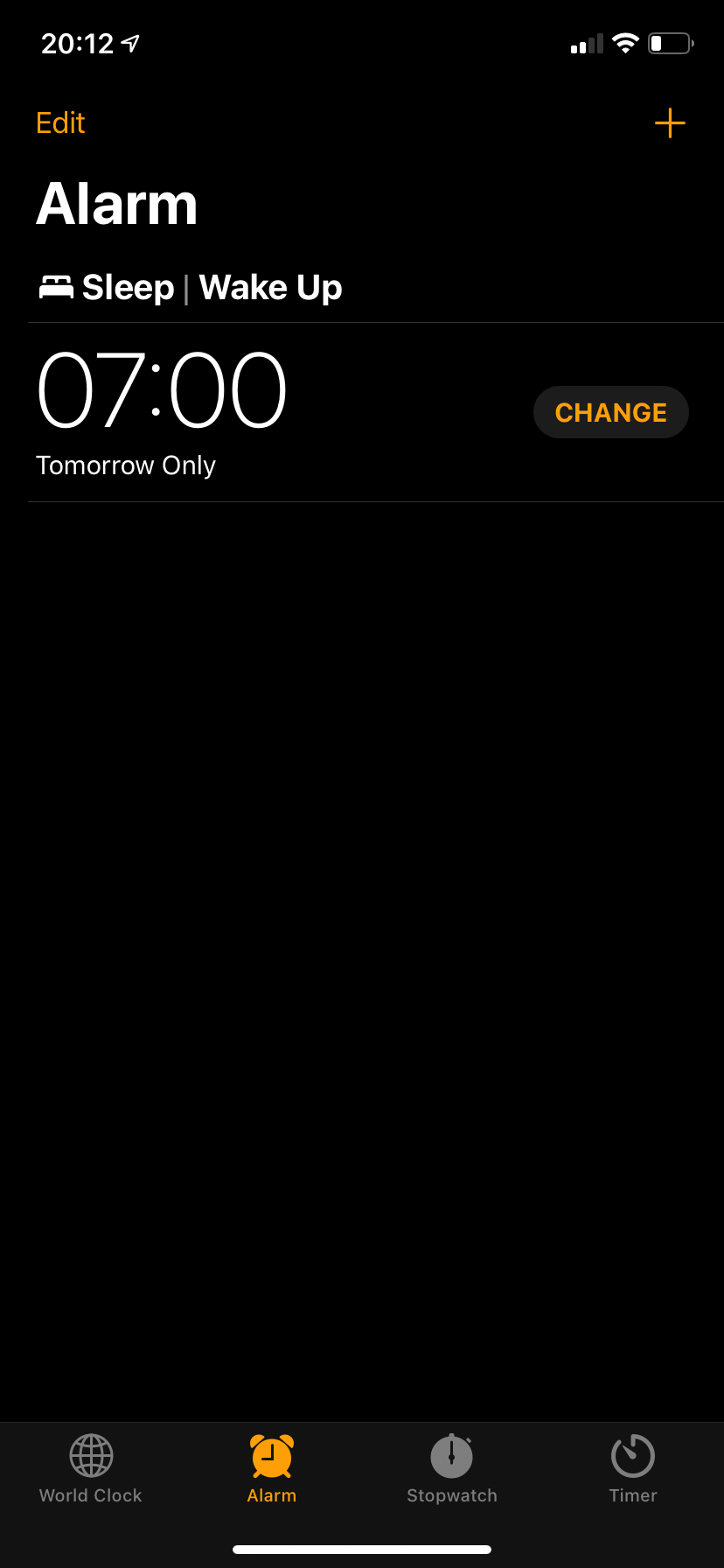The screenshot displays the user interface of an alarm-setting application on a mobile device, likely a smartphone or tablet. Central to the image is the alarm time, which is currently set for 7:00 AM. Adjacent to the alarm time is a prominent orange button, enabling users to easily modify the wake-up time with a simple tap. 

The app interface offers two distinct options: one for setting an alarm at bedtime (“Sleep”) and another for scheduling shorter rest periods or naps (“Wake Up”). Indicators within the screenshot reveal the device is connected to Wi-Fi and has a low battery level, with the current device time displayed as 20:12 (8:12 PM). 

The intuitive design of the app ensures users can effortlessly adjust their alarms for overnight sleep or short naps, evidenced by the active orange icon. The concise layout and clear instructions make it straightforward to navigate and manage alarm settings.